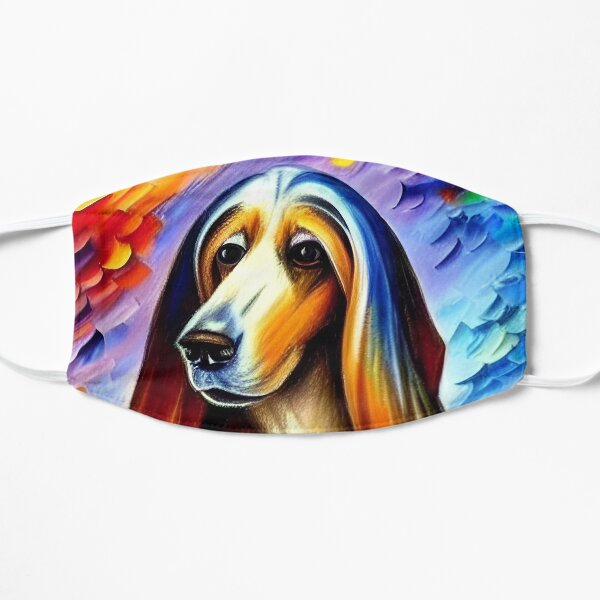This detailed image showcases a face mask, similar to those worn during the COVID-19 pandemic, positioned against a pristine white background. The mask, with its white elastic loops stretched to either side, reveals a vivid and intricate design featuring an Afghan hound at its center. The dog's visage is rendered in a style reminiscent of colored pencil art, with a serene expression and eyes gazing into the distance. Its elongated snout and silky, flowing ears, which cascade down like luxurious hair, are depicted in a blend of colors: white with hints of lighter golden brown, dark orange, and even an overlay of reddish and bluish hues. The dog's ears especially evoke an image of long, dyed hair, adding a surreal, almost ethereal quality to its appearance.

The backdrop of the mask boasts a radiant gradient of colors, transitioning from warm tones of orange, red, and yellow on the left to cooler shades of purple and blue towards the right. There are also touches of green interspersed throughout. This vibrant and colorful spectrum enhances the artistic appeal of the mask, making it an eye-catching piece. The combination of the Afghan hound's detailed depiction and the dynamic, multicolored background creates a product that is both visually captivating and richly detailed, perfect for use in a promotional or sales setting.